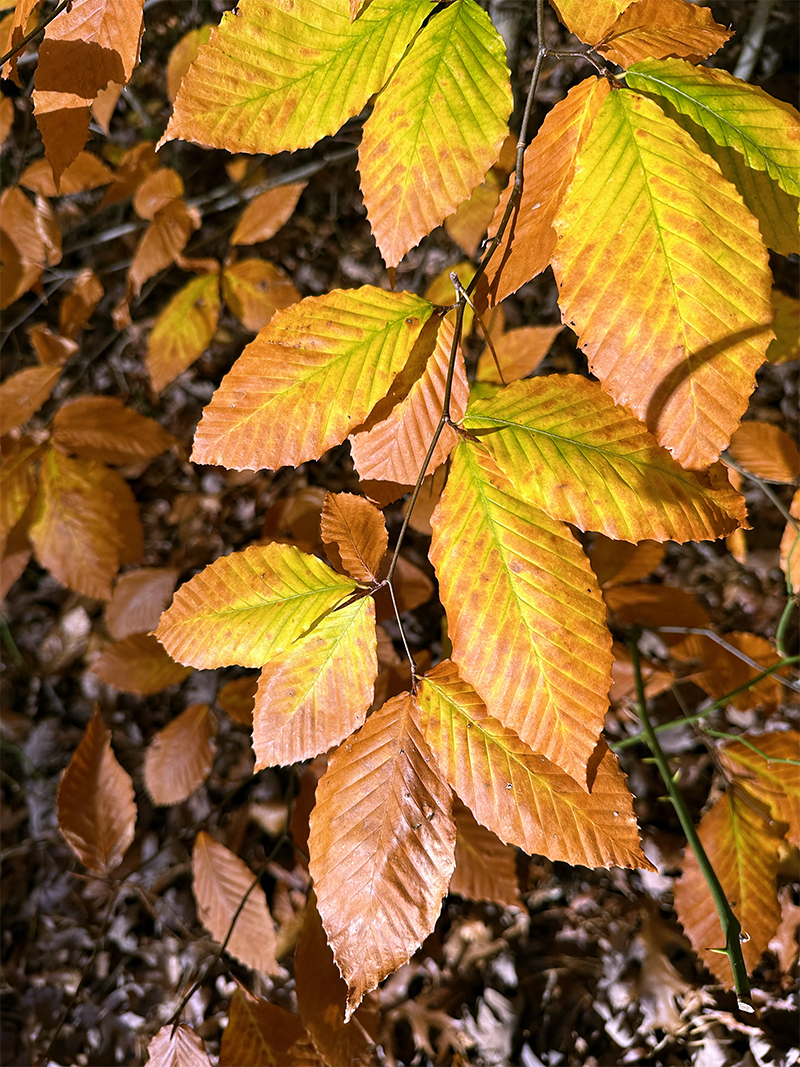This close-up photograph captures the intricate beauty of a tree or shrub in the midst of autumn. Thin, brown branches adorned with clusters of two or three diamond-shaped, serrated leaves hang low towards the ground. The leaves are predominantly orange and yellow, signifying the fall season, with lingering hints of green along their central veins. The ground below, visible in the background, is covered with dirt and scattered old leaves, adding to the seasonal ambiance. A few rocks and a thorned vine are also visible in the distance, creating a textured, natural backdrop. The composition draws focus to the foreground leaves while subtly revealing clusters of similar leaves, slightly blurred, further beyond.